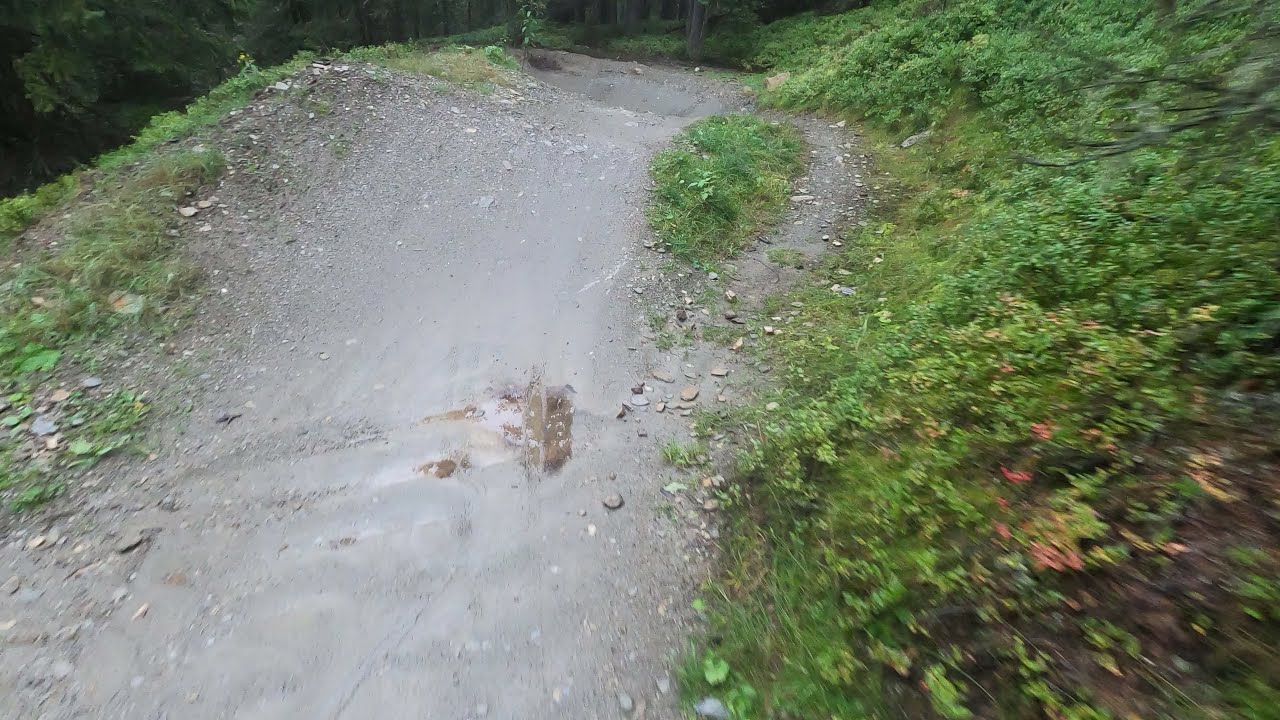The photograph captures a damp, grayish dirt path that begins at the bottom left corner and meanders up to the top of the frame, flanked by lush vegetation. The path, wide enough to possibly be a dirt bike trail, appears muddy and wet, indicative of recent rain. On the right side, an abundance of greenery, including moss, grass, and bushes, rises along a slight incline. The left side features more plants, but the terrain drops off, suggesting the presence of a low hill or a cliff-like edge. The blurry appearance of the trees and bushes hints that the photo was taken while in motion, adding a dynamic feel. Scattered stones and a few red leaves are visible at the bottom right corner, but the landscape is predominantly varied shades of green, exuding a dense, jungle-like atmosphere. The scene is closely framed, focusing solely on the path and adjacent foliage, enveloping the viewer in the intimate, verdant setting.